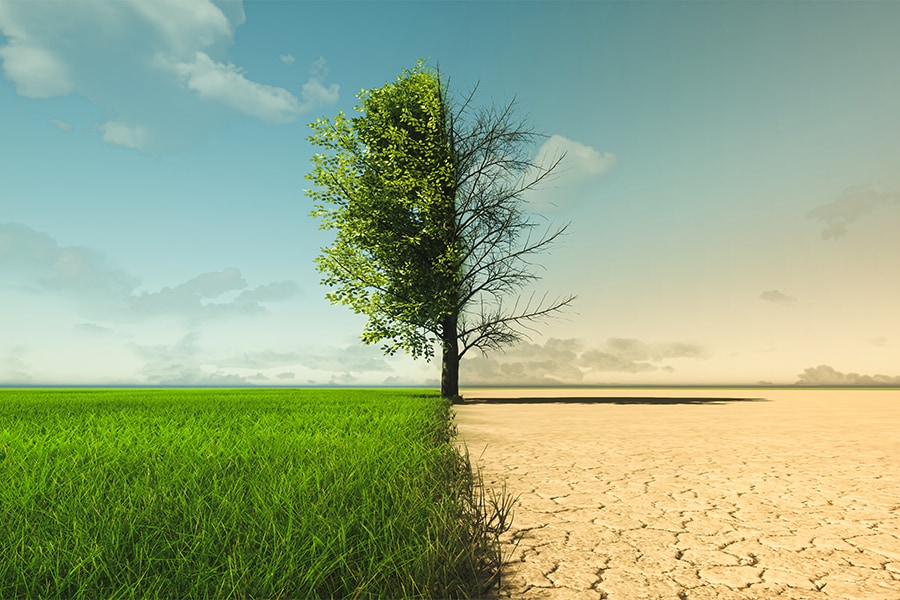The image is a striking representation of contrasting environments, possibly illustrating the impacts of climate change. The scene is meticulously split down the middle, featuring a single tree at the center as the focal point. The left side is a picturesque, vibrant landscape, characterized by lush, well-manicured green grass extending into the distance. The sky above this side is a clear blue with a few wispy white clouds, enhancing the overall sense of vitality and health. The left half of the tree is bursting with green leaves, symbolizing life and abundance.

In stark contrast, the right side of the image portrays a barren, desolate environment. The ground is dry and cracked, resembling an arid desert that has seen no rain. The sky on this side is a dusty grayish-blue, perhaps indicating a scene affected by dust storms or pollution. The right half of the tree mirrors this lifelessness, with bare branches devoid of any foliage, starkly contrasting with its lush counterpart on the left.

The entire composition seems to visually depict a "before and after" scenario, highlighting the stark differences between fertile, healthy land and dried, parched earth. This powerful image underscores the potential consequences of environmental neglect or climate change, creating a vivid, visual dichotomy between life and desolation.